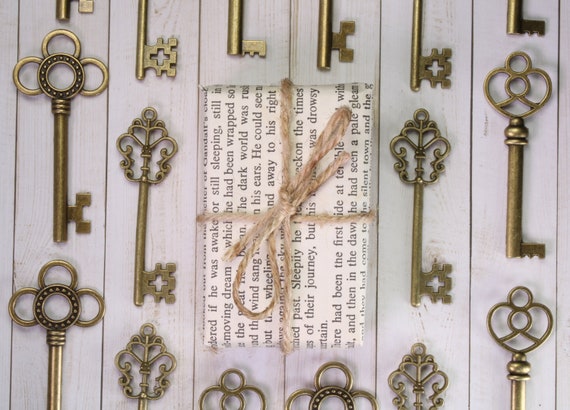This photograph, in a portrait layout format, showcases an artistic arrangement of various ornate, old-fashioned brass keys laid out in perfectly vertical formation on a pale gray wood plank surface with narrow black lines defining the gaps between the boards. The planks run vertically across the image. In total, the photograph reveals four fully visible keys: the top left key features a circular design with three partial circles merging into it, leading down to a two-prong shaft; the second key, to its right and lower, has an intricate top and a more notched shaft; directly opposite this, on the other side of the central object, another key mirrors this ornate style; the fourth, situated above this one, showcases a rounded top, followed by a heart-like frame encircling another circle, a thicker shaft, and several notches to the right. Moreover, the image includes partially visible keys, with the bottoms of six keys at the top edge and the tops of six keys at the bottom edge of the frame.

Central to this meticulous arrangement is a square object wrapped in a piece of paper resembling a page from a book or newspaper. The text on the paper is oriented vertically, requiring a 90-degree turn to be read, with the top of the text towards the left and the bottom towards the right. This wrapped object is neatly tied with brown twine in a crisscross pattern, with a bow in the center, adding a rustic and mysterious touch to the composition. This intricate and detailed scene blends historical elegance with modern artistic aesthetics.